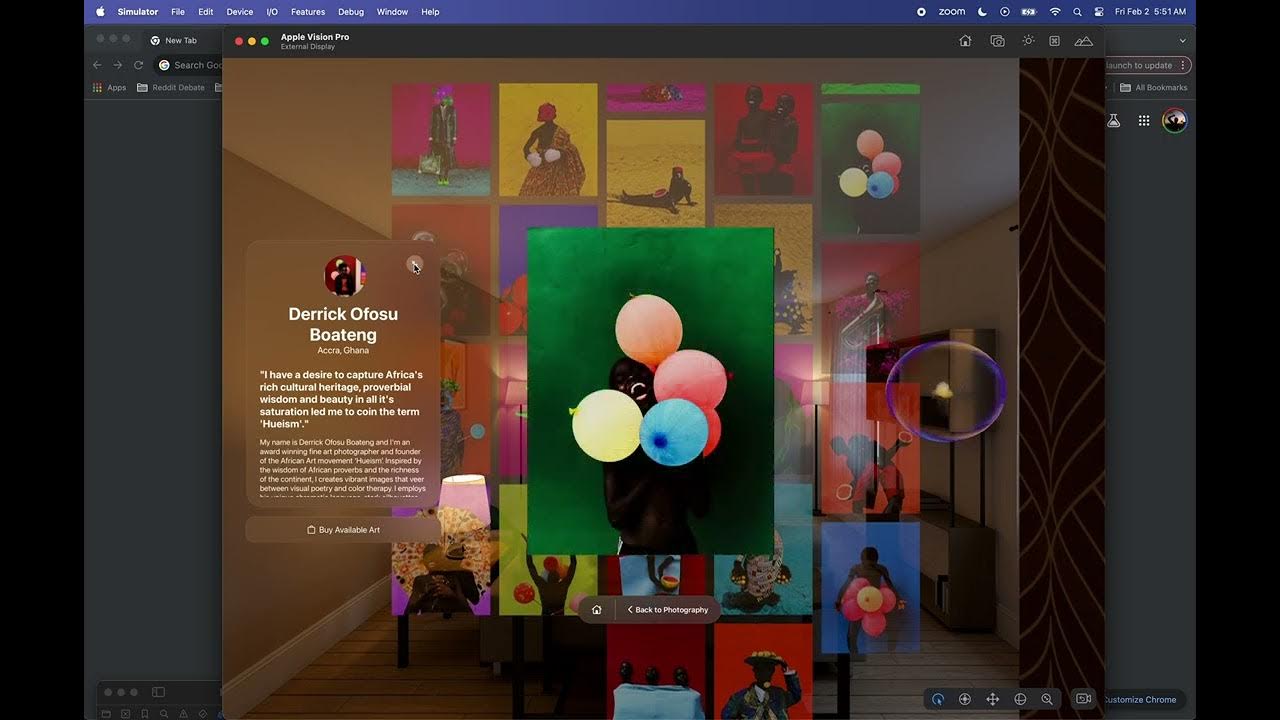This image is a detailed screenshot of a computer monitor displaying a web page. The web page prominently features a large central rectangular photo with a dark emerald green background, where an African American person is depicted laughing with their head tilted back, showcasing bright white teeth. Surrounding the person are multiple colorful balloons—two red, one orange, one blue, and one yellow—framing their face. The monitor itself displays a web browser with a black and blue interface, including a recognizable menu on the left and standard computer icons, including the time, on the right.

To the left of the photo, towards the middle of the screen, there is a block of text identifying the artist: Derek Afosu-Botang from Accra, Ghana. The accompanying text provides a brief biography, mentioning that Derek Afosu-Botang is an award-winning fine art photographer and the founder of the African Art Movement. In the background, the web page is adorned with several other pieces of art, suggesting that these images are part of a gallery where each piece can likely be expanded for more detailed viewing.